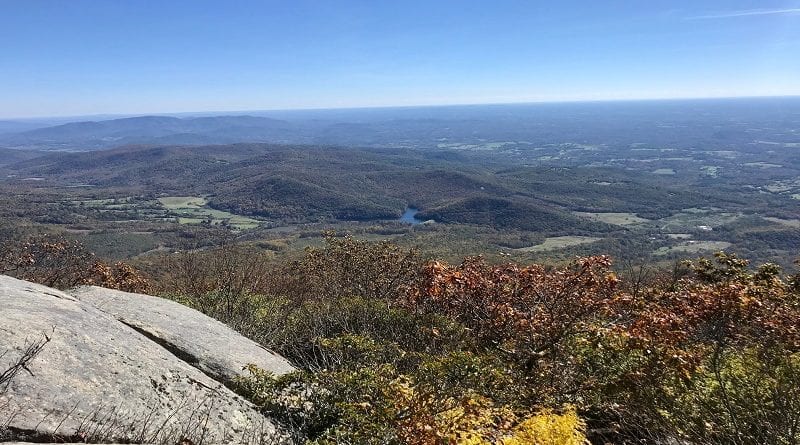The image captures a stunning daytime vista from the peak of an iconic mountain in the Blue Ridge range of Virginia. Taken from a vantage point atop flat, expansive rocks, the view reveals an expansive valley filled with lush greenery that stretches endlessly into the distance. Foregrounded by vibrant autumnal foliage in shades of orange, yellow, and green, the scene is framed by a deep blue sky. Amid the rolling hills, a small body of water, possibly a river or reservoir, glistens at the center. Scattered rocks and a mixture of tree tops cover the hillside, with more of the Blue Ridge Mountains forming a hazy, distant skyline. No signs of urban life—only the natural beauty of grass, trees, and untouched wilderness.